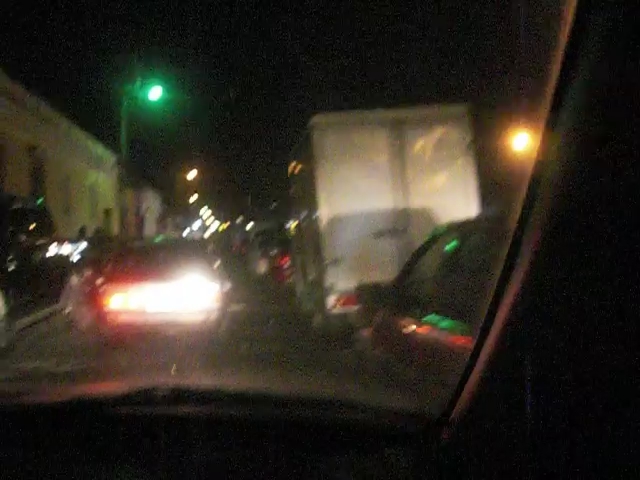A blurry nighttime photograph taken from inside a vehicle traveling on a crowded street. Illuminated by streetlights, the bright red taillights of the vehicle directly ahead dominate the foreground, emphasizing the bumper-to-bumper traffic. To the right, the image captures the partial front of a sedan in the neighboring lane, followed by a large semi-truck positioned ahead of it. The left lane, which the vehicle is occupying, reveals a series of cars extending into the distance. The sidewalks flanking the street are faintly visible, hinting at the silhouettes of pedestrians. A combination of green and yellow street lamps cast an ambient glow, contributing to the urban nightscape.